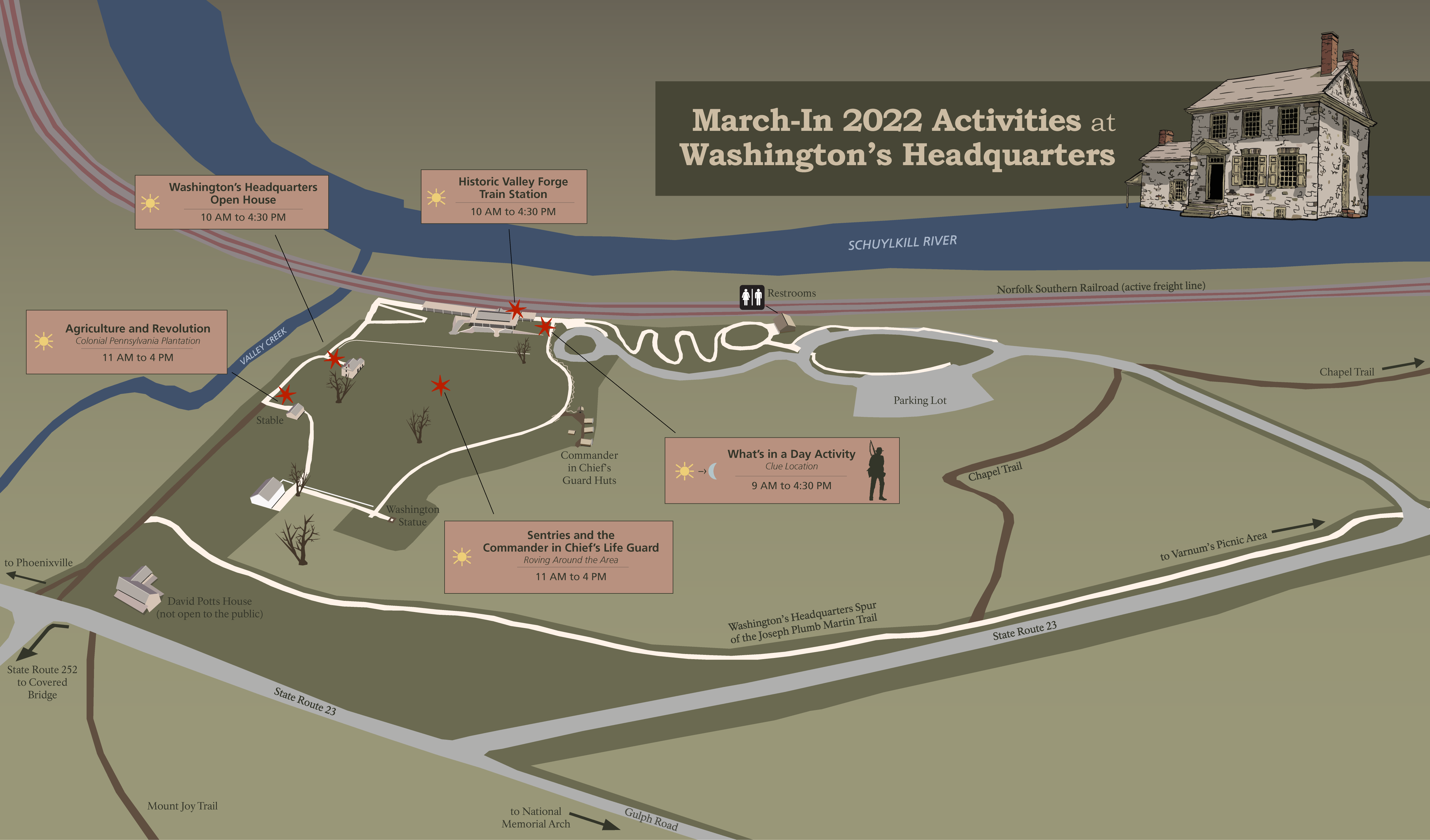The image is a detailed map likely found in a textbook or court case, illustrating the Washington's Headquarters area. The map is primarily green, with shades of olive and light pale green. In the top right corner, an olive green bar with tan text reads "March-End 2022 Activities at Washington's Headquarters." Beside this text, there’s an image of an old house with green stains and two chimneys.

The map features several roads highlighted in gray, including State Route 23 and Mount Joy Trail, which leads to Phoenixville. A prominent blue river flows through the top of the map, identified as the Sculchey-Kill River, and another labeled Valley Creek. Red stars mark significant locations, while brown rectangles provide descriptions that are difficult to read due to their tiny text. The map also includes various symbols such as roundabouts, restrooms, and directional arrows guiding how to leave the area.